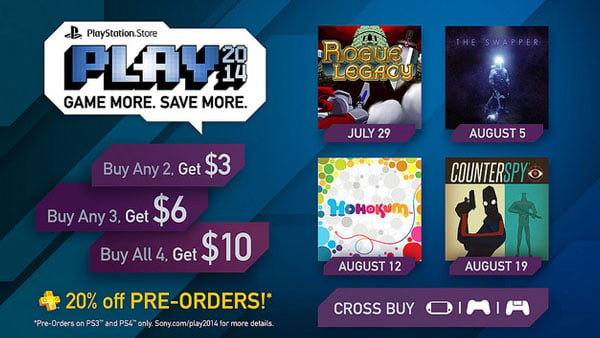The image features a website advertisement with a dark blue background adorned with lighter blue vertical diagonal stripes. In the top left-hand corner, a white box contains prominent text. It reads "PlayStation Store Play" in large blue letters, followed by "2014: Game More, Save More" in purple blocks. Below, additional offers are detailed in similarly colored blocks: "Buy any two, get $3," "Buy any three, get $6," and "Buy all four, get $10." A prominent yellow cross below these offers advertises "20% off pre-orders," with a note underneath clarifying "Pre-orders on PS3 and PS4 only. Visit Sony.com/play2014 for more details."

On the right-hand side, there are four images showcasing upcoming game releases:
1. "Rogue Legacy" with a release date of July 29.
2. "The Swapper" releasing on August 5.
3. "HOHOKUM" available August 12.
4. "CounterSpy" set for August 19.

Beneath these images, a purple box with the text "Cross-Buy" appears, accompanied by icons representing a game console, a computer, and gaming controllers.